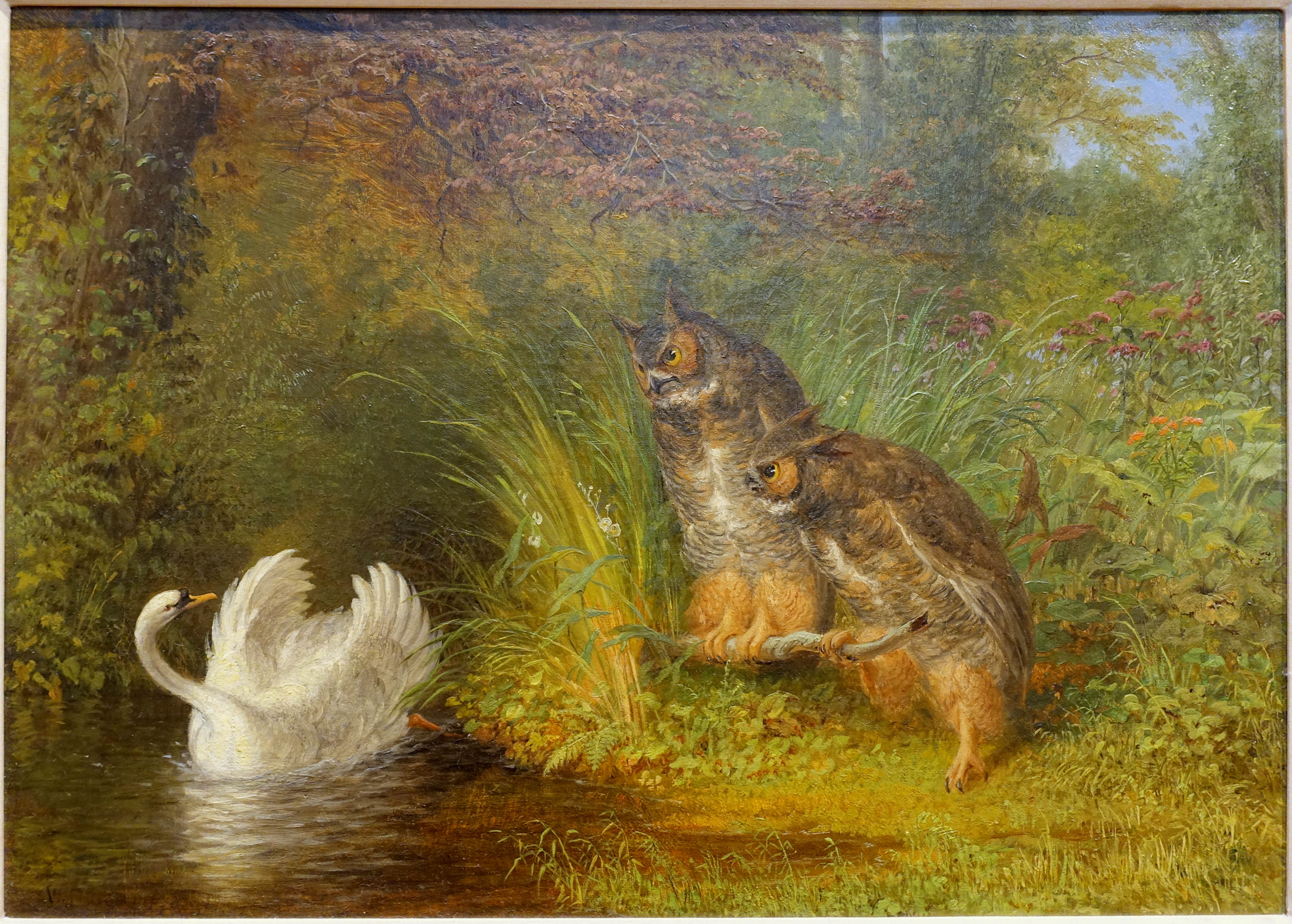In this detailed painting of a lively nature setting, two brown owls are perched on a branch on the right side, appearing to intently watch a distressed white swan in the murky, brownish water on the left. The owls, with their light golden-brown and light brown feathers, seem almost as if they're bullying the swan, who is flapping its wings and looking back at them with a curved neck, displaying a black mark on its nose. The scene is abundant with lush greenery, featuring grass, flowers, and various shrubs in deep auburn and vibrant green hues. Overarching branches and the tops of trees frame the image, with a hint of a light blue sky peeking through the top right corner. The vibrant foliage and the serene yet tense interaction between the owls and the swan create a captivating focal point.